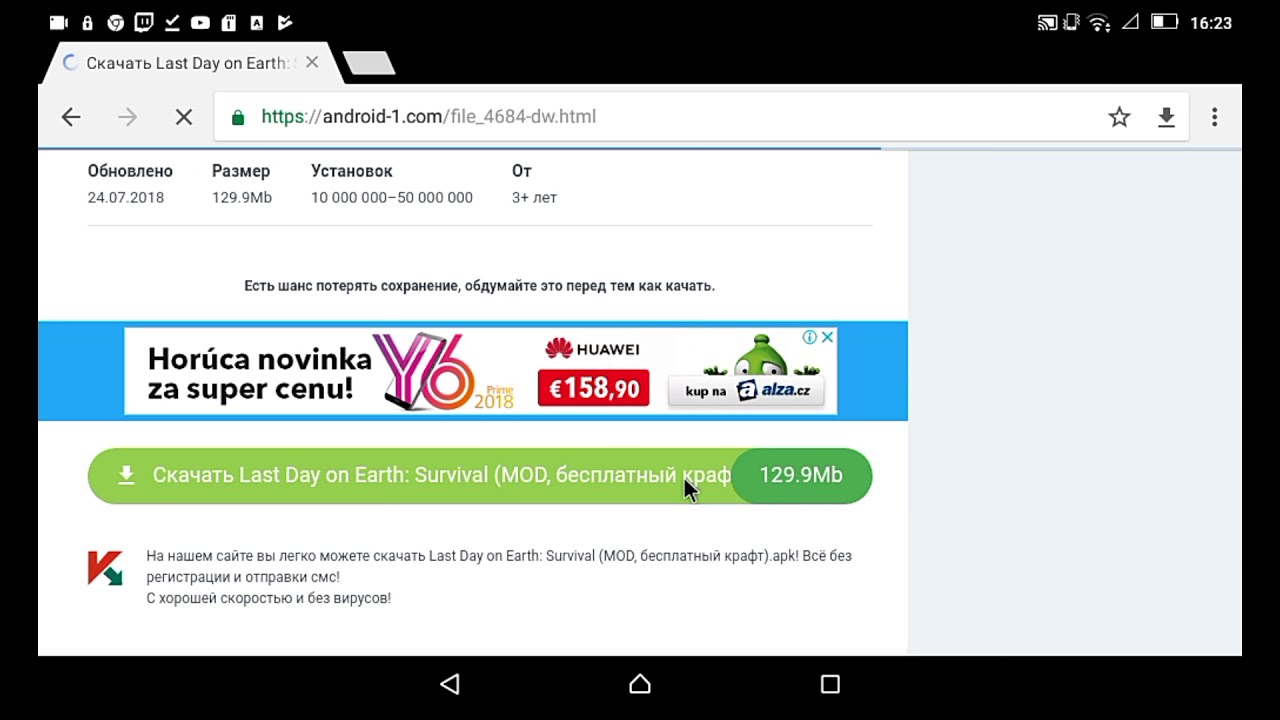The screenshot depicts a webpage primarily in a foreign language, visibly accessible at "https://android-1.com/file4684-DW.html" with a gray-themed layout and a highlighted address bar. The page headline reads "Last Day on Earth" and the subtitle indicates "Last Day on Earth Survival" accompanied by a file size notation of "129.9 MB." Dominating the left side of the webpage is a large white square, possibly an image or placeholder. A navigation bar at the top is followed by a colorful advertisement against a blue stripe, featuring multi-colored text in red, purple, green, white, and yellow. Below this advertisement, a green stripe with white writing 'Last Day on Earth: Survival' is noticeable, under which black text continues in the non-English language. The screen also displays common computer interface elements like volume, internet connectivity, battery level indicators, and a clock showing "16:23."